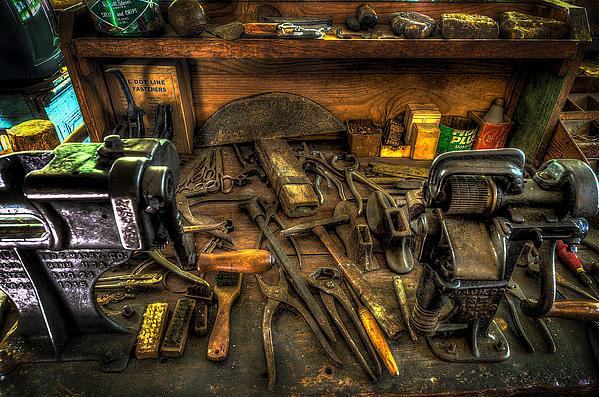This incredibly detailed and realistic drawing of a workshop scene depicts a well-worn, rustic wooden workbench cluttered with an array of old and heavily rusted tools. The workbench, possibly set in a garage or a workroom, features several tools such as wrenches, pliers, hammers—including a ball-peen hammer and a mallet—a screwdriver, and multiple vice grips scattered across its surface. Prominently, there are clusters of mini clamps, hammer heads, and brushes—both steel and non-steel bristled—neatly lined up. A large iron anvil with a slight shine occupies the bottom left corner, reflecting light from an unknown source. Mounted machinery, solidly built from steel, adds to the vintage, rugged aesthetic of the scene. Adding to the depth, a rich brown wooden shelf in the background holds unidentifiable items, giving an impression of a workstation frequented long ago but now lying untouched, evoking a sense of abandonment and history.